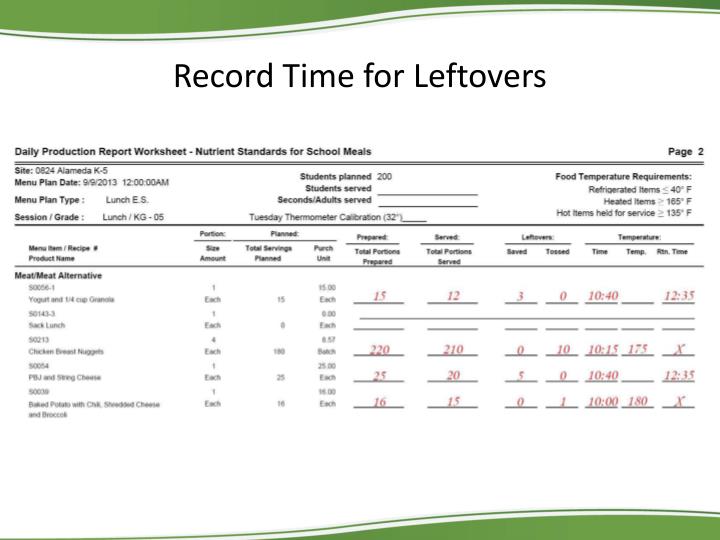The image depicts a rectangular worksheet set against a plain white background, measuring approximately four inches tall by six inches wide. At the top and bottom, the worksheet features a decorative green border that forms a wave pattern, wider on the left and tapering to a thin strip on the right, accented with an additional green pinstripe.

Centered at the top in bold black print, the title reads "Record Time for Leftovers," followed by "Daily Production Report Worksheet - Nutrient Standards for School Meals" on the left and "Page 2" on the far right. Below this header, two pinstripes extend horizontally across the page. The worksheet pertains to the Alameda K-5 school site with details such as the menu plan date of 9-9-2013 at 12 a.m. and is related to lunch for grades K-5.

The worksheet is divided into several sections, each bordered by black lines and containing various details and columns. The detailed sections include information such as students planned (200), students served, and food temperature requirements. Specific columns list data pertaining to projected service, servings, leftovers, and temperatures recorded in red ink.

The lower portion of the worksheet includes detailed instructions and sections for menu items, recipe product names, portion sizes, total servings planned and prepared, and the status of leftovers. The left side specifically mentions categories like "Meat/Meat Alternatives," while the right side provides quantitative data in red ink, detailing figures like prepared servings and temperatures.

Overall, the worksheet is a comprehensive report for tracking daily meal production and compliance with nutrient standards, complete with precise layouts for recording critical data points required for school meal planning and execution.